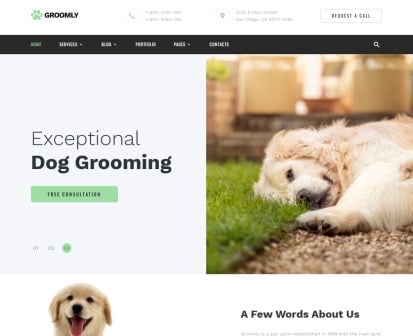The image appears to be a screenshot of a website for a dog grooming service named "Groomly." At the top, there is a green paw print logo with the text "Groomly" in black. Below this, there's a white banner featuring a gray phone icon and several phone numbers alongside a green location pin and an address; both the phone numbers and the address are too blurry to be read clearly.

Continuing down the page, there is a black menu bar with white text and dropdown menus, including a white magnifying glass icon for search functionality. Below this menu bar lies a gray box containing the text "Exceptional Dog Grooming" in black. Alongside this box is a green button that says "Free Consultation" in black text. Additionally, there are three icons within this gray box, one of which is circled in green.

Adjacent to the gray box, the image displays a dog with shaggy blonde fur resting its head on green grass, with one paw placed on tan pebbles. In the blurry background, a tan house is partially visible.

Beneath this section, the webpage features another descriptive box with the heading "A Few Words About Us" in black, followed by some grey textual content. On the other side, underneath the gray box, is an image of a blonde dog with a pink tongue hanging out, a black nose, dark eyes, and floppy ears.

While the image is somewhat zoomed out, making finer details challenging to discern, the overall visual quality is good.